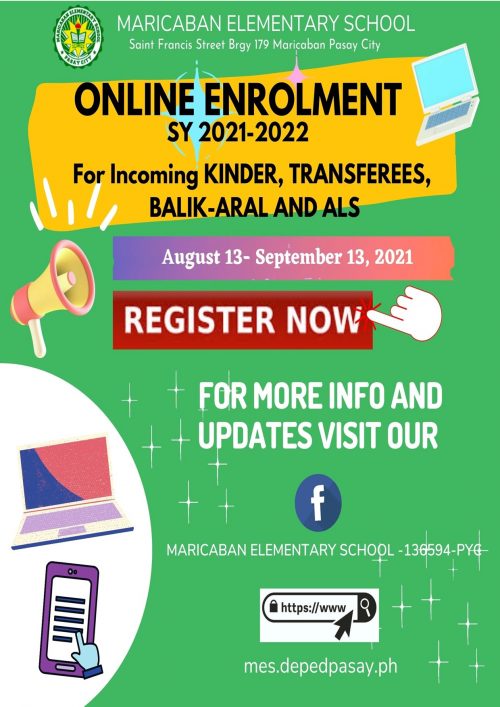**Banner Ad for Marikabian Elementary School Online Enrollment**

The image is a vertical rectangular banner ad, approximately twice as tall as it is wide, with a light green background.

**Header:**
At the very top, the text is written in white capital letters stating:
- **MARIKABIAN ELEMENTARY SCHOOL**
- **ST. FRANCIS STREET**
- **BRGY 179 MARICABAN**
- **PASAY CITY**

**Left Side:**
On the left side of the banner, there is the school's coat of arms, featuring a central yellow color with an image of a book, enclosed in a white circle, set against a gold-yellow background.

**Main Content:**
The banner prominently displays a rectangle, slightly irregular in shape, with the following details in black capital letters:
- **ONLINE ENROLLMENT**
- **S.Y. 2021-2022**
- **For Incoming Kinder, Transferees, **Balik-Aral NALS**

Accompanying this text is a simple drawing of a laptop computer on the right side of this section, indicating online registration. 

**Dates:**
The enrollment dates are displayed within a vertically split rectangle, purple on the left and light pink on the right. The text reads:
- **AUGUST 13th TO SEPTEMBER 13th, 2021**

**Call to Action:**
Beneath this, in a red rectangle with white letters:
- **REGISTER NOW**

**Additional Information:**
Against the green background, with white font, the banner provides further instructions:
- **For More Info and Updates, Visit Our**

Followed by the Facebook logo, a blue circle with a white letter "F".

**Footer:**
At the very bottom of the banner, it lists the web address:
- **mes.depedpasay.ph**

This detailed banner ad is designed to inform and prompt parents and guardians to register their children for the upcoming school year at Marikabian Elementary School through an online enrollment process.